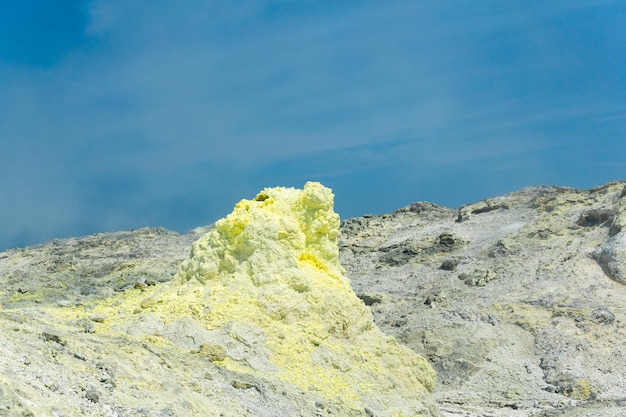The photograph captures a stunning nature scene showcasing a striking contrast between the azure, mostly clear sky, and the rugged, rocky landscape below. The sky, a very bright blue with a few thin, stretched-out clouds scattered faintly, serves as a serene backdrop to the main focus of the image - the rocky cliff face. This rough, gray terrain is adorned with craters and indentations, giving it a textured, moon-like appearance. The landscape slopes downward from the taller right side to the shorter left side, creating a dynamic visual interest. In the center foreground, amidst the gray rocks, there lies a peculiar mound of yellow, powdery rocks. This yellow formation appears unnatural and stands out vividly against the gray, extending slightly upwards, hinting at being either remnants of shoveled snow, dumped chemicals, or some other anomaly. The vivid contrast between the natural rock and the inexplicable yellow pile adds an intriguing element to the otherwise serene natural beauty of the scene.